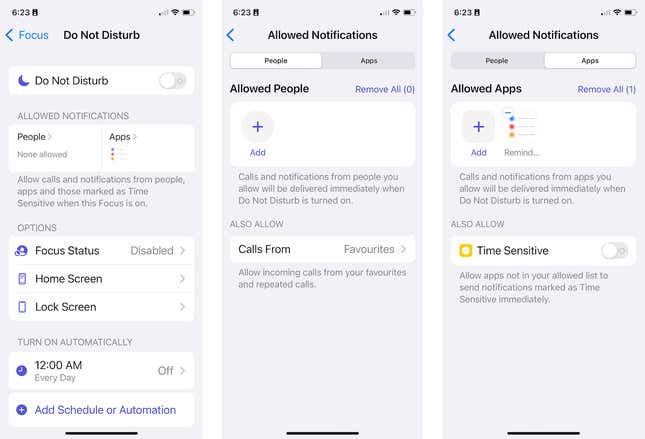The image is divided into three distinct sections, each appearing as a screenshot from a smartphone interface that depicts various settings related to the "Do Not Disturb" feature.

**Section 1: Overview Settings**
- **Top Header:**
  - A time indicator showing "6:23."
  - The word “Focus” accompanied by an arrow pointing to the left.
  - A toggle option labeled “Do Not Disturb,” with a moon icon beside it.
- **Options Below:**
  - "Allow Notifications" section.
  - "Focus Status" with a label indicating it is disabled.
  - "Home Screen" with an arrow pointing right.
  - "Lock Screen" with an arrow pointing right.
  - A schedule setting showing "12 a.m. Every Day" with the status being off and an option to "Add Schedule or Automation."

**Section 2: People Notifications**
- **Header:**
  - A section titled "Allowed Notifications."
  - Subsection for "People" with an "Apps" option next to it.
- **Content:**
  - "Allowed People" in bold text.
  - A plus symbol next to "Add."
  - Explanation: “Calls and notifications from people you allow will be delivered immediately when Do Not Disturb is on.”

**Section 3: Apps Notifications**
- **Header:**
  - Continuation of "Allowed Notifications."
  - "People" and "Apps" sections.
- **Content:**
  - Header "Allowed Apps" with a plus sign next to "Add."
  - An option labeled "Remind" with three circles above it.
  - Explanation: “Calls and notifications from apps you allow will be delivered immediately when Do Not Disturb is on.”
  - An option for "Time Sensitive" with a yellow square and a clock icon beside it.

Overall, the image comprehensively showcases the various settings and customization options available for managing notifications during the "Do Not Disturb" mode on a smartphone.